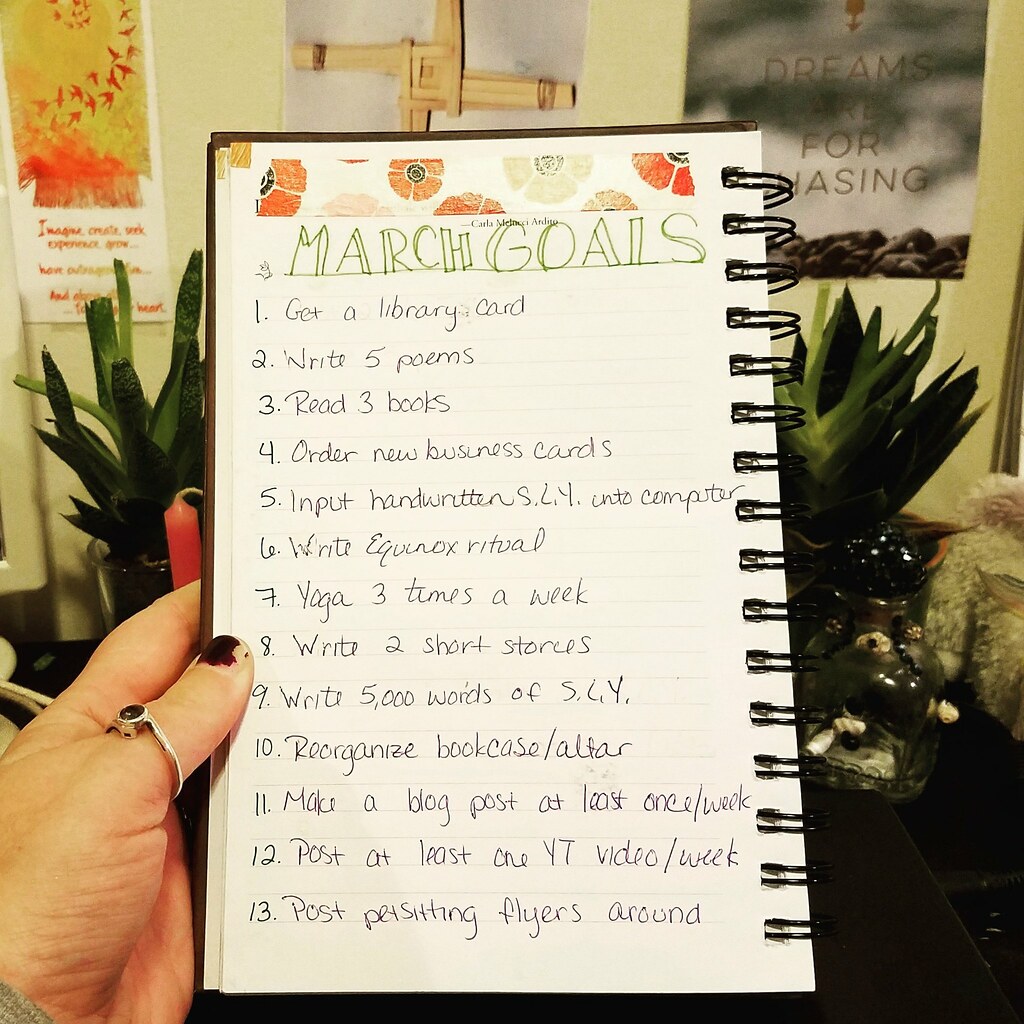This large square image captures a photograph taken indoors, prominently featuring a small spiral notebook held by a person's hand in the lower left-hand corner. The hand, adorned with a thumb ring set with a dark gemstone, displays chipped dark red nail polish on the thumb. The black spirals of the notebook are visible on the right side. Inside the notebook, the top of the page is decorated with a flowered border, and the title "March Goals" is written in large green letters. The page lists goals numbered one through thirteen: 1. Get a library card, 2. Write five poems, 3. Read three books, 4. Order new business cards, 5. Input handwritten SLY into the computer, 6. Write an Equinox ritual, 7. Practice yoga three times a week, 8. Write two short stories, 9. Write 5,000 words of SLY, 10. Reorganize the bookcase/altar, 11. Make a blog post at least once a week, 12. Post at least one YouTube video per week, 13. Post pet-sitting flyers around. In the background, details of a room are visible, including green leaves of potted plants on a desk and posters on the wall, accentuating the personal indoor setting. The color palette includes touches of yellow, orange, red, white, green, tan, gray, and pink.